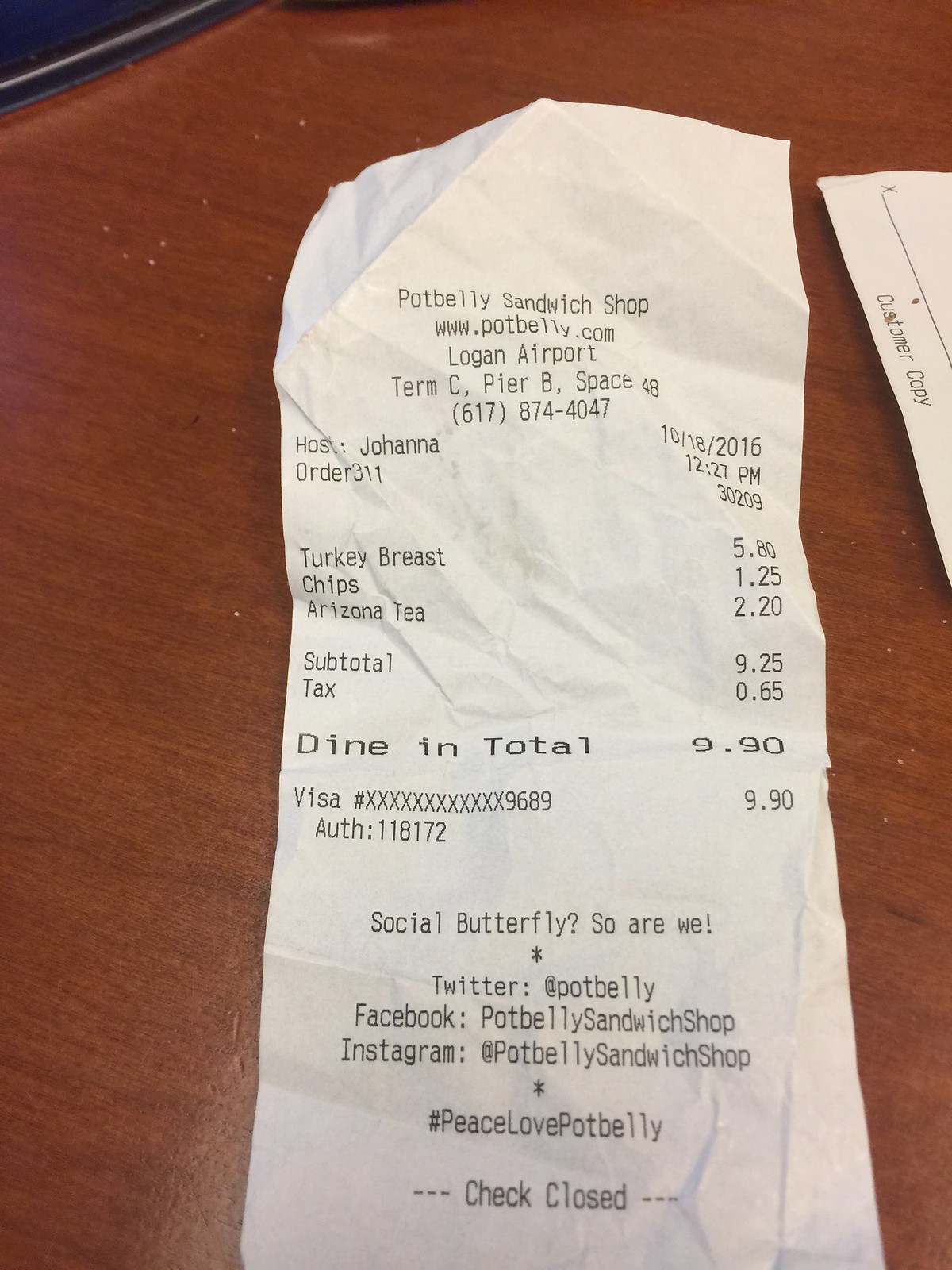A slightly crinkled and folded, white receipt lies on a wooden table. The top of the receipt proudly displays "Potbelly Sandwich Shop" along with their website, www.potbelly.com. This particular receipt is from their Logan Airport location, specifically Terminal C, Pier B. The phone number listed is 617-874-4042. The host who attended to the customer was named Johanna, and the receipt is dated October 18, 2016, at 12:27 p.m., with the order number 311.

The customer ordered a turkey breast sandwich priced at $5.80, a bag of chips costing $1.25, and an Arizona tea for $2.20. The subtotal for the meal came to $9.25, and after adding $0.65 in tax, the total amount due was $9.90. A Visa card with the last four digits 9689 was used for the payment. 

Towards the bottom of the receipt, there is a friendly social media prompt: "Social Butterfly? So are we," followed by the social media icons for Twitter, Facebook, and Instagram, encouraging customers to connect using the hashtag #PeaceLovePotbelly. Finally, the receipt concludes with the words "check closed."